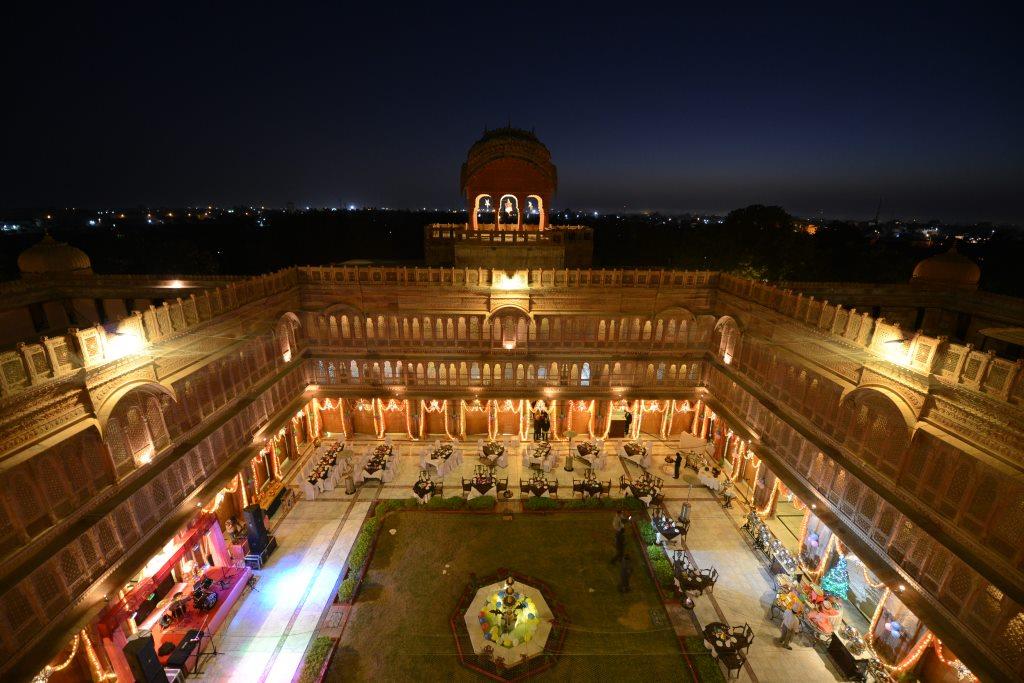The image features a stunning nighttime view of a potentially famous building, possibly located in Rome. This multi-level, gold-tinged tan building surrounds a bustling courtyard filled with details. A central rectangular patch of vibrant grass is home to a picturesque fountain, possibly adorned with balloons. Surrounding this lively space is a pinkish stage and numerous tables and chairs, indicating an event is underway. The night sky forms a serene backdrop, contrasting with the well-lit scene below. Spotlights enhance the courtyard's colorful ambiance, illuminating the lawn with hues of pink, green, blue, and white. Notable features include three bells in the building's prominent tower and elegant windows providing glimpses inside. The atmosphere is festive, with decorative greenery and vivid lighting adding to the scene’s charm, suggesting it might be around Christmas time.